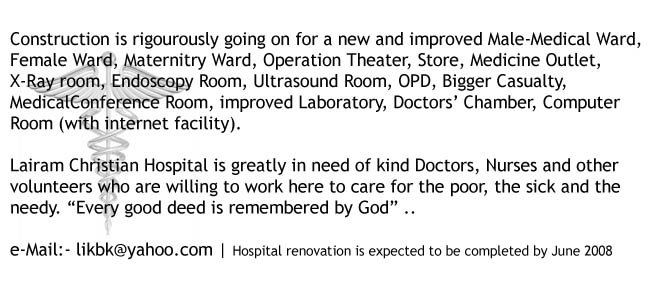The image features plain black text against a white background with a subtle watermark of a caduceus symbol—a staff with two intertwined snakes and wings—positioned on the left side, partially overlapping the text. The message, which takes up the entirety of the image, reads from the upper left corner with no borders or indents. It states:

"Construction is rigorously going on for a new and improved male medical ward, female ward, maternity ward, operation theater, store, medicine outlet, X-ray room, endoscopy room, ultrasound room, OPD, bigger casualty, medical conference room, improved laboratory, doctor's chamber, computer room with internet facility."

The subsequent paragraph highlights the dire need of Laram Christian Hospital for dedicated doctors, nurses, and other volunteers committed to caring for the poor, sick, and needy. It emphasizes, "Every good deed is remembered by God." 

At the bottom, across the line from left to right, it lists an email—email-likbk@yahoo.com—and indicates that the hospital renovation is expected to be completed by June 2008.